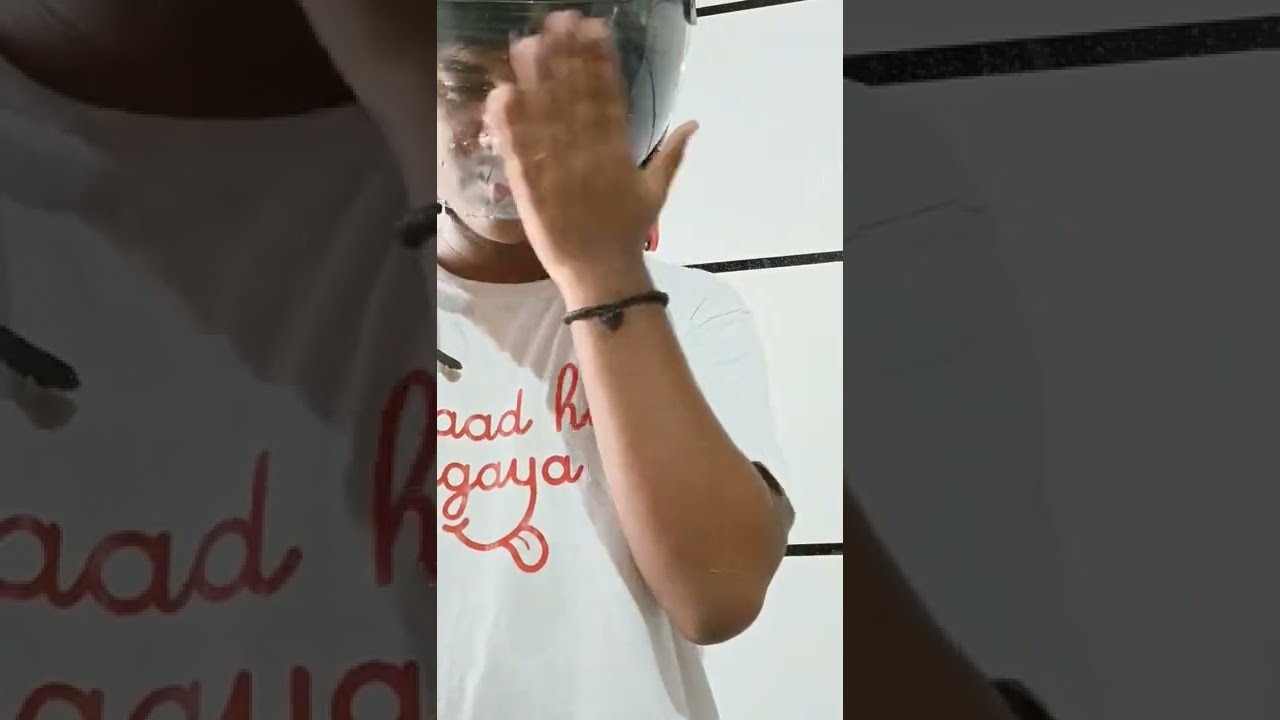The image showcases a man standing against a white backdrop with three horizontal black lines. He is wearing a white t-shirt featuring the letters "AAD" in red font and a graphical design that includes a letter "Y" with a stylized, tongue-like tail. The man has darker skin and is potentially of Indian descent. His left arm is raised, with his hand fully extended and partially covering his face. His hand appears blurry due to motion. He is wearing a black, corded bracelet with a black heart detail. The man also dons a black motorcycle crash helmet. His face has some substance smeared on it, and he is looking down with a closed mouth. The image is a vertical cell phone style photograph, with the left and right edges duplicated, zoomed in, and faded. The camera is angled slightly upwards from the lower chest level of the man.